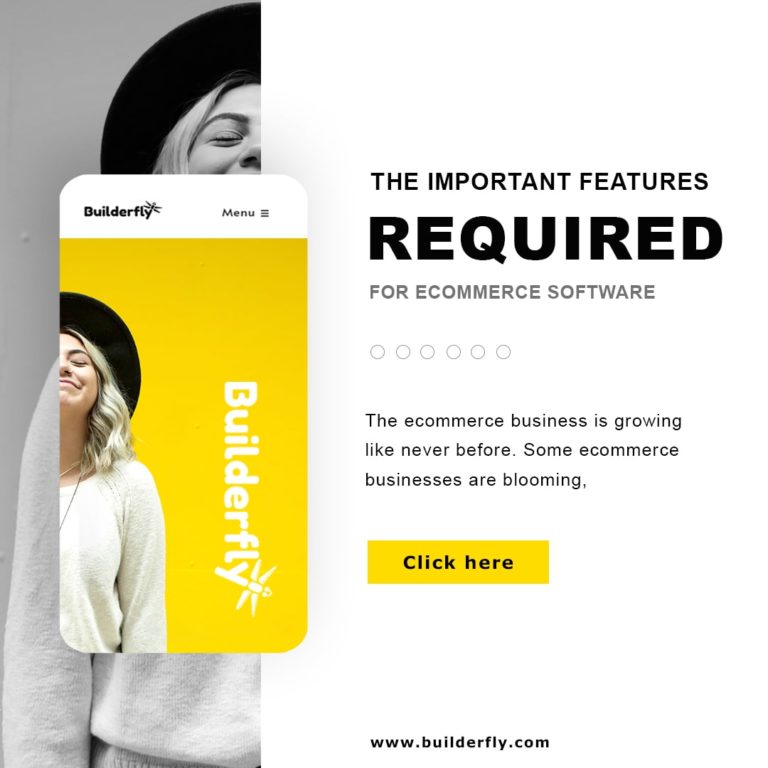The image appears to be a screen capture of an advertisement. On one side, there is a black-and-white photo of a woman wearing a black hat in the background. Overlaid on this is a colorized version of the same photo, showing the woman with blonde hair, her head tilted upwards, a partial smile on her face, and her eyes closed. She is wearing a white sweater and a black hat.

At the top of the image, there is a white bar with the text "Builderfly" in black, followed by the word "Menu." Below this bar, the background turns yellow, prominently featuring the colorized version of the woman’s photo. To the side of this image, "Builderfly" is written in white text.

Further down, there is black text that reads, "The important features required for ecommerce software." Directly beneath this text are six gray dots arranged in a row. Below the dots, more black text states, "The e-commerce business is growing like never before. Some e-commerce businesses are blooming." Following this, there is a gold box with the words "Click Here" in bold black font. At the bottom of the image, the URL "www.builderfly.com" is displayed.

The overall image quality is clear, with a user-friendly font. Notably, the letter "Y" in "Builderfly" includes a small icon resembling a dragonfly. There are no additional elements of note.